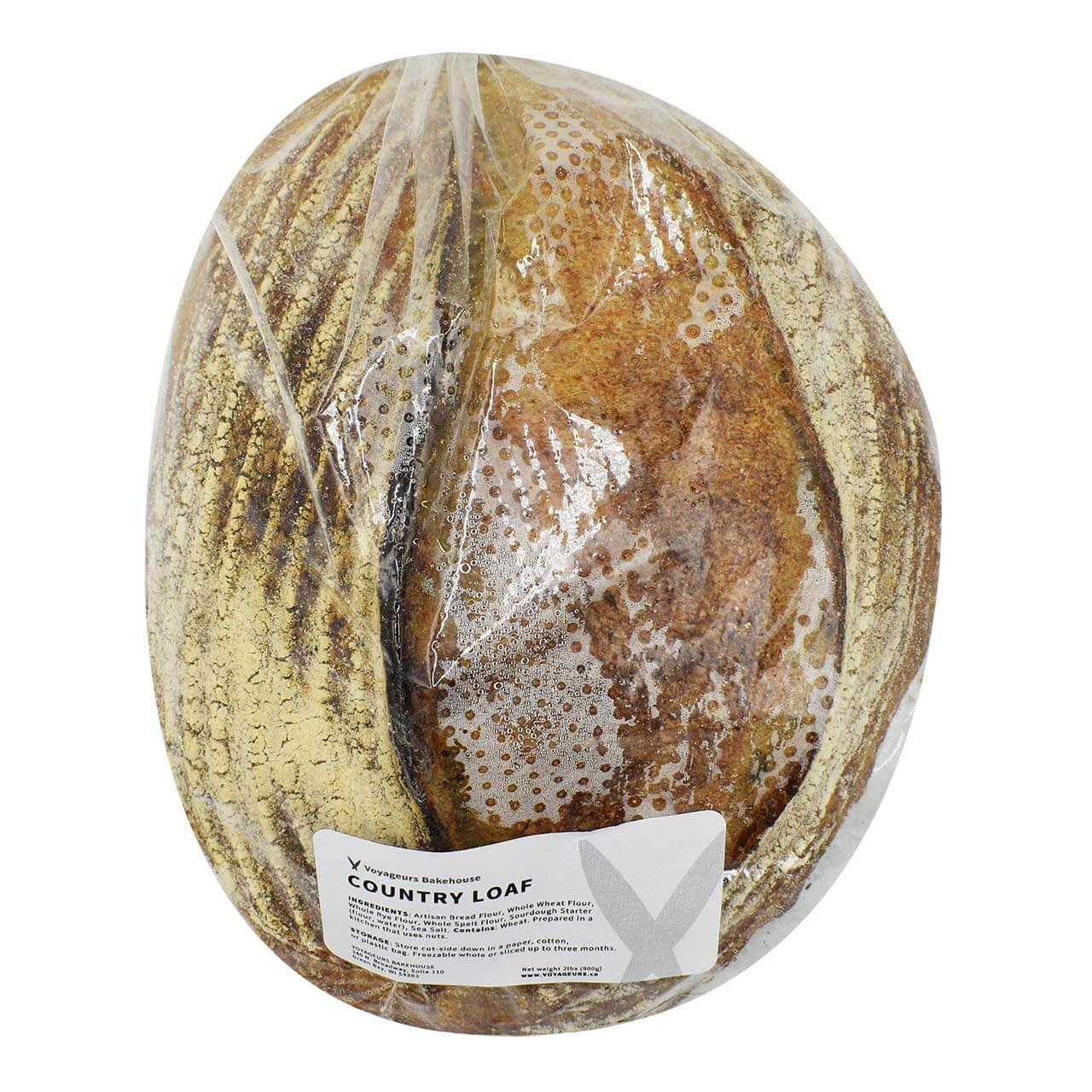This photograph features a round, air-sealed loaf of bread lying against a pure white background. The bread, which has the shape and heft reminiscent of a small basketball, is tightly wrapped in clear plastic, capturing the loaf's distinct surface texture. There is noticeable condensation within the plastic wrapping, particularly concentrated in the center and forming small dots of moisture. The loaf itself has a varied color palette: the left side displays a thicker layer of yellowish-tan dusting over dark, ridge-like stripes, while the right side mirrors this design with a thinner dusting. Nestled between these two sections, the central part of the bread bears a richer brown hue akin to a muffin's surface, accentuated with darker, ridged swaths.

Attached to the front of the plastic wrap is a white label with rounded corners. The label's design includes a small black X-shaped logo in the top left corner, next to the text "Voyager's Bakehouse." Beneath this, boldly printed in larger black text, are the words "Country Loaf." Further down the label, the ingredients are listed: "Artisan bread flour, whole wheat flour, whole rye flour, whole spelt flour, sourdough starter (flour, water), sea salt. Contains wheat. Prepared in a kitchen that uses nuts." Lastly, the label provides storage instructions: "Store cut side down in a paper, cotton, or plastic bag. Freezable whole or sliced up to three months." Two small blocks of illegible text are seen at the bottom corners of the label, completing the detailed, wholesome presentation of this artisan bread product.